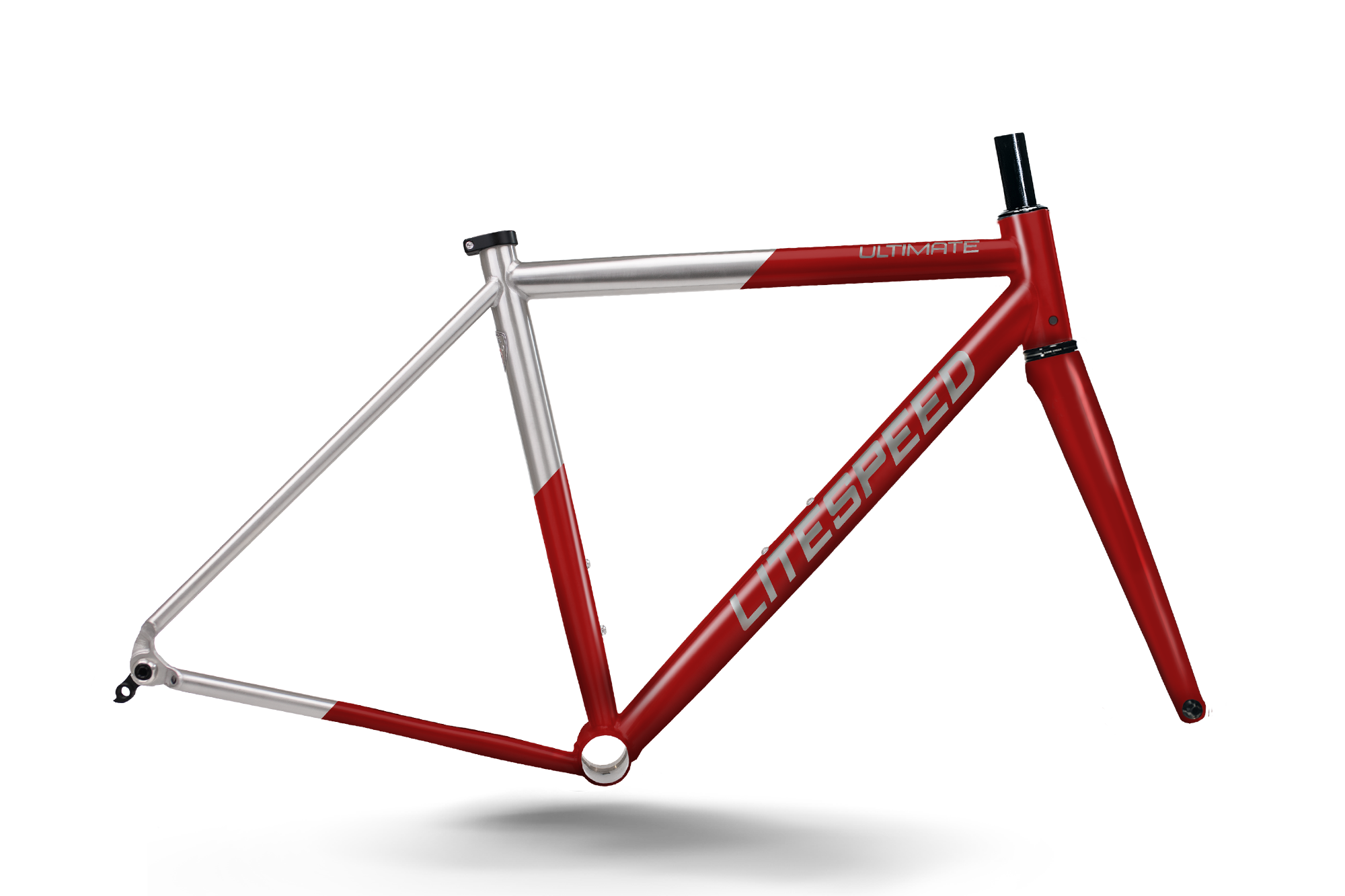The image showcases a floating bike frame against a white background, casting a light gray circular shadow beneath it. The frame, predominantly red and silver, is a diamond shape formed by several connected bars without any attached components like tires or seats. The right section includes a slightly bent vertical red bar with a small black rod protruding from the top. Extending horizontally to the left is a half-red, half-silver bar with the word "ULTIMATE" inscribed in gray, all caps. From there, another red bar angles downward to the left bearing the word "LIGHTSPEED" written in large gray all caps. Connecting these is a red and silver vertical bar with a black cap on top, culminating in a silver bar that extends towards the lower left and then redirects back to the right, forming a triangular section with a circular cutout. The overall design features a glossy finish, emphasizing the sleekness and intricate construction of the bike frame.